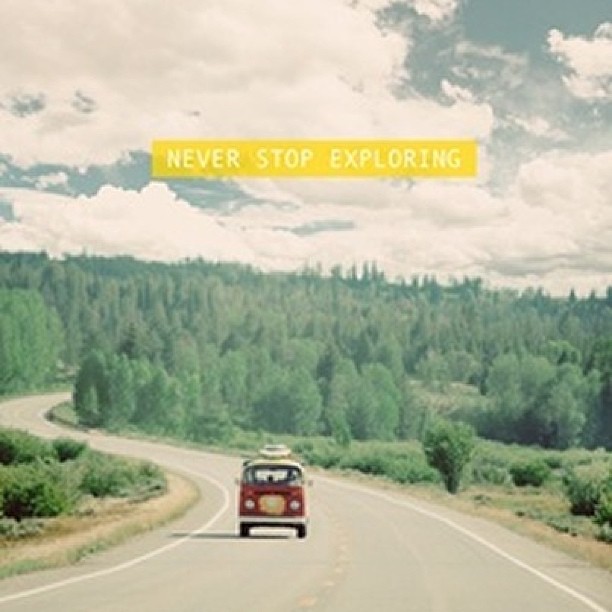The image captures a nostalgic, adventure-themed photograph of a winding, single-lane country road, characterized by a mix of asphalt and earthy, brown dirt. Dominating the bottom center of the frame is a red Volkswagen minibus with a white top and an attachment for luggage, ascending the road and adding a quaint, vintage charm to the scene. The road is flanked by an array of trees, shrubs, and grass, giving way to a lush green forest that stretches towards the horizon, creating a serene and picturesque rural landscape. The sky, occupying the upper portion of the image, is filled with fluffy white clouds against a vibrant blue backdrop, further enhancing the idyllic and adventurous spirit of the setting. Emblazoned across the top of the image in a bold, yellow rectangular box with white text are the words "Never Stop Exploring," suggesting a call to adventure and road trips. The overall atmosphere suggests an outdoor, daytime scene, reminiscent of vintage travel advertisements often shared on social media to evoke a sense of nostalgia and wanderlust.